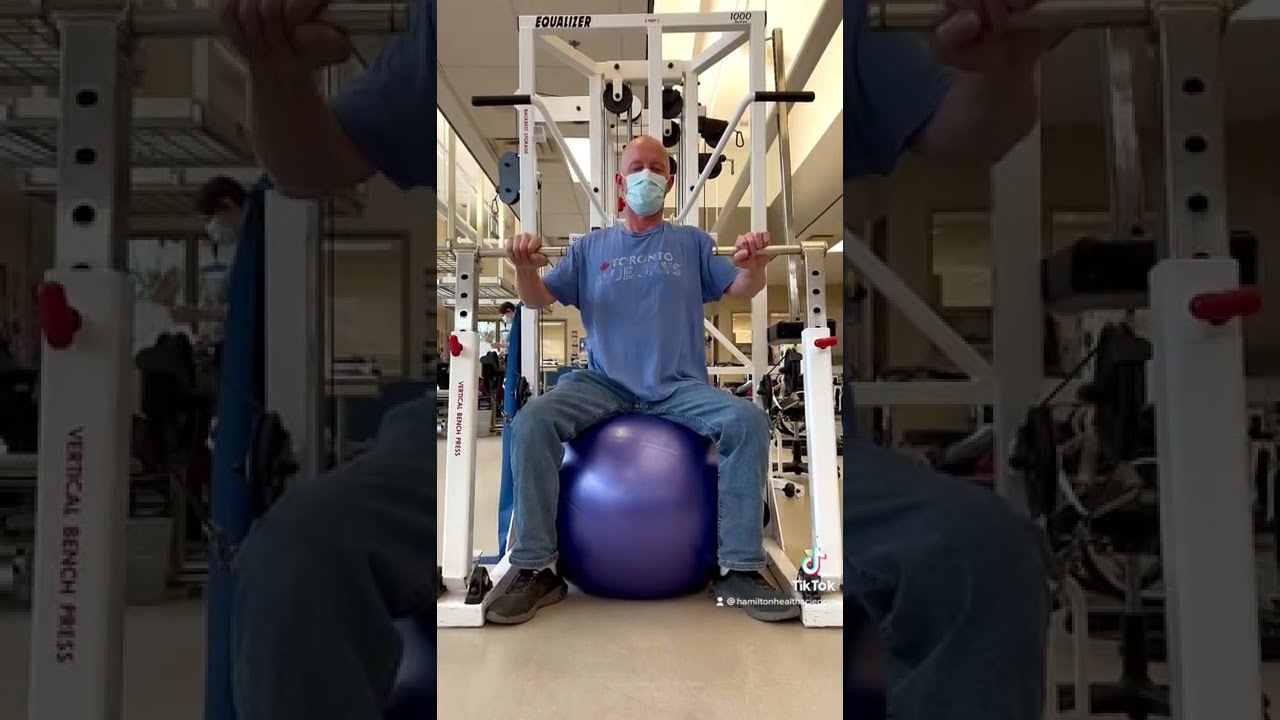In a brightly lit gym, a Caucasian man sits on a dark purple exercise ball in front of a white Vertical Bench Press machine. The man, who appears to have a bald head, is wearing a light blue t-shirt with the words "Toronto Blue Jays" in white, blue jeans, black sneakers, and a blue medical face mask covering his nose and mouth. His arms are extended to either side, gripping the metallic handles of the exercise machine at about waist height. The machine features black lettering reading "Equalizer" at the top left and "1000" at the top right, while also displaying the TikTok logo and a username in the bottom right. Visible in the background is a door and various gym equipment, with a monochrome filter adding a dim border to the left and right sides of the image. There's another individual faintly visible in the distance.